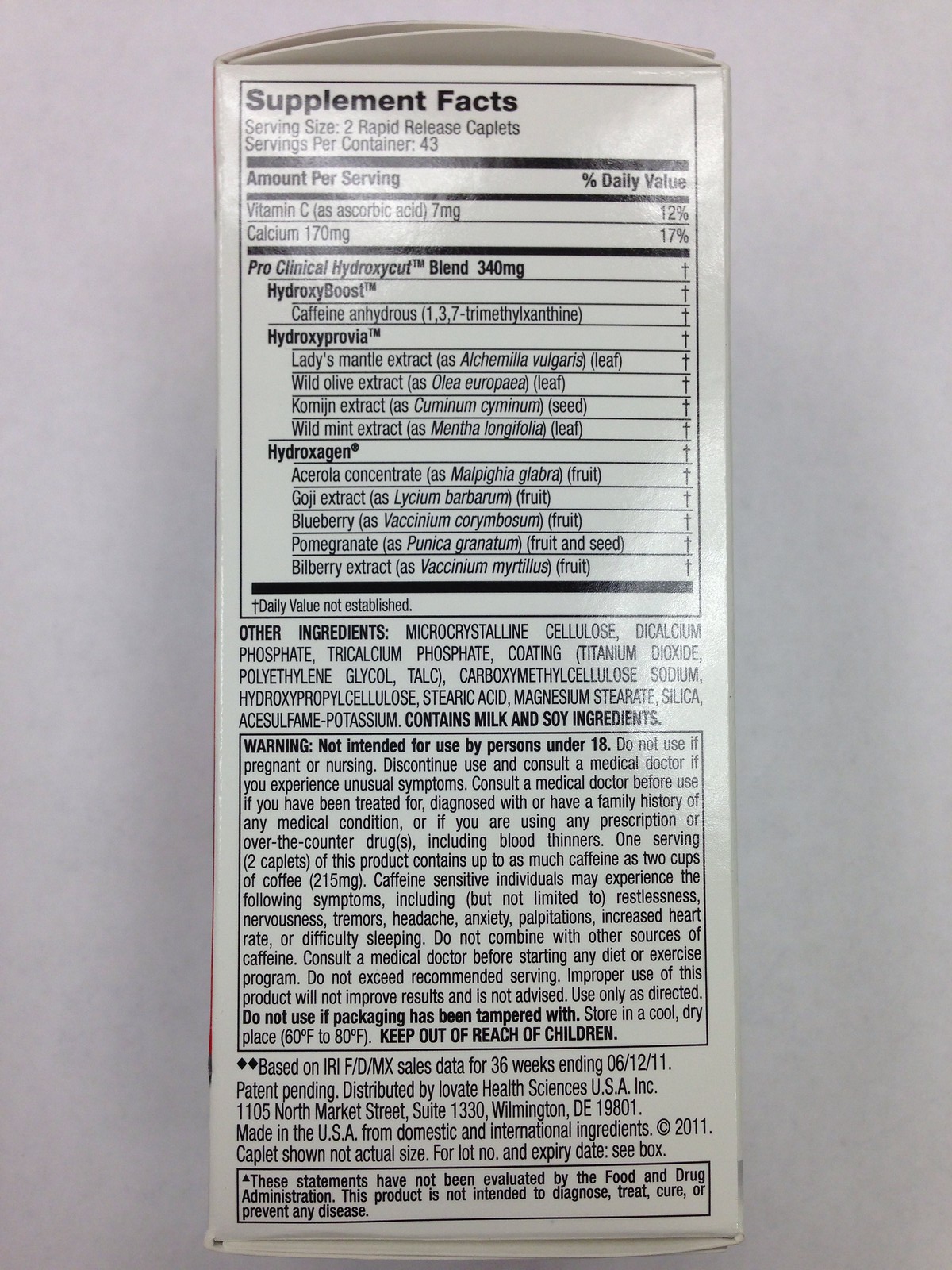This is a photograph of a box of dietary supplements turned on its side, prominently displaying the nutritional labels. At the top of the label, the text "Supplement Facts" is printed in large, bold letters. Surrounding this section is a neatly defined box. Inside this box, it specifies "Serving Size: 2 Rapid Release Caplets" and "Servings Per Container: 43." The information is presented in two columns: one titled "Amount Per Serving" and the other "Percent Daily Value." These columns list the quantities for Vitamin C and Calcium.

Below the "Supplement Facts" box, there is a section labeled "Other Ingredients," followed by a separate "Warning" box with additional cautionary information for consumers. The overall design of the label is organized and clear, making it easy to read the detailed nutritional information and warnings displayed on the box.